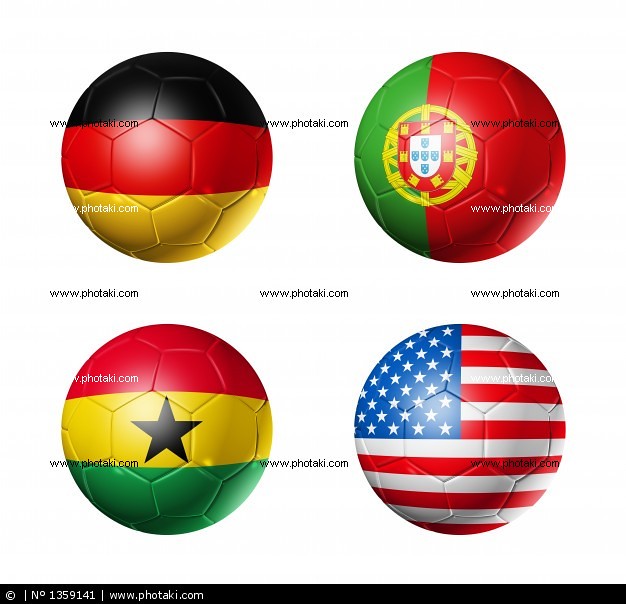The image is a computer-generated graphic depicting four soccer balls, each adorned with different national flags. The soccer balls are arranged in a square format with prominent pentagon and hexagon panels typical of their design. The upper left ball features the German flag with black, red, and yellow stripes. The upper right ball displays the Portuguese flag, characterized by its distinctive red and green halves plus an intricate crest that includes blue, white, and yellow elements. The bottom left ball represents Ghana with its colors: red top, yellow middle featuring a black star, and green bottom. The bottom right ball showcases the American flag, with its stars in the upper left section and red and white stripes. The image is watermarked with "www.fotaki.com" multiple times, indicating it is likely a stock photo, and includes a copyright notice at the bottom with the number 139141 and the website www.fotaki.com.